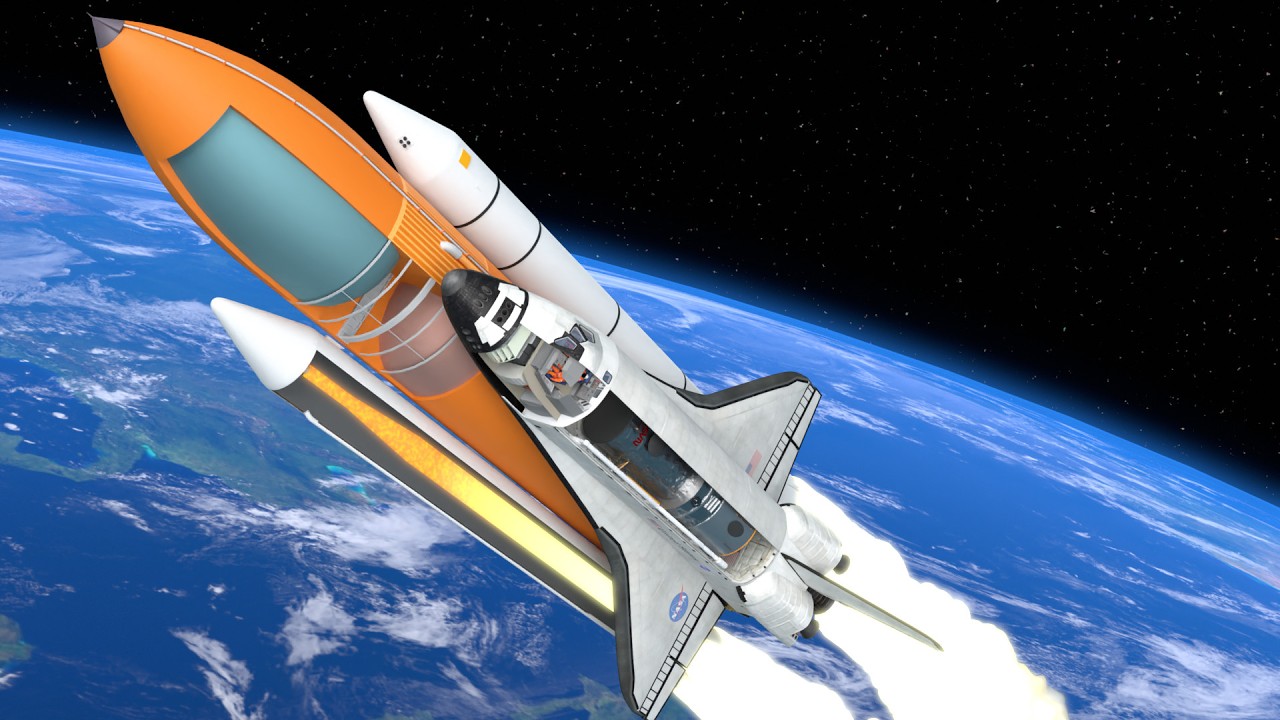This image is a detailed artistic rendering of a space shuttle launch in a landscape orientation. It features a modern NASA space shuttle mounted on a large orange booster rocket, accompanied by smaller white rockets. The launch appears to be in its initial stages, with fire and smoke emanating from the bottom of the rockets, propelling the spacecraft from the lower right towards the upper left. The scene is set against a backdrop of Earth, visible as a blue expanse with clouds, albeit zoomed out. The image incorporates both 3D graphic elements and a bit of a cutaway view that reveals the interior seating for passengers and the cargo bay inside the shuttle. The caption "Space Shuttle Launch" is prominently displayed, with "Space Shuttle" in white text and "Launch" in a larger yellow font, emphasizing the event depicted. Wispy clouds streak the sky, adding to the dynamic sense of motion and ascent. The portrayal evokes historical NASA missions, potentially alluding to iconic shuttles like the Challenger.